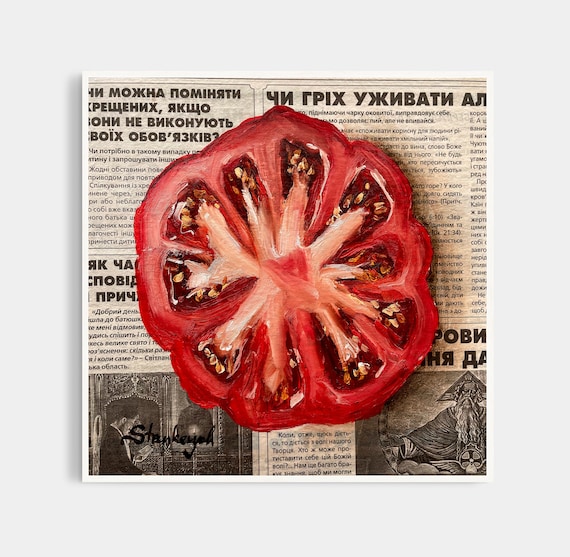This image features a striking painting of a tomato slice, rendered in various shades of red with a lighter-colored center highlighting its seeds, resembling a tomato slice that might adorn a hamburger. The painted tomato is superimposed on a black-and-white newspaper clipping in what appears to be an Eastern European language, potentially Ukrainian or Russian. The clipping includes distinct headers in bold and several black-and-white images, laid out in traditional paragraph format. The painting itself is meticulously detailed, capturing the essence of the tomato's texture and coloration. The bottom left corner of the piece bears the artist's signature, which reads "STANKEYOH." The entire composition is set against a plain white background, ensuring the painted tomato and newspaper snippet remain the focal points of the image.